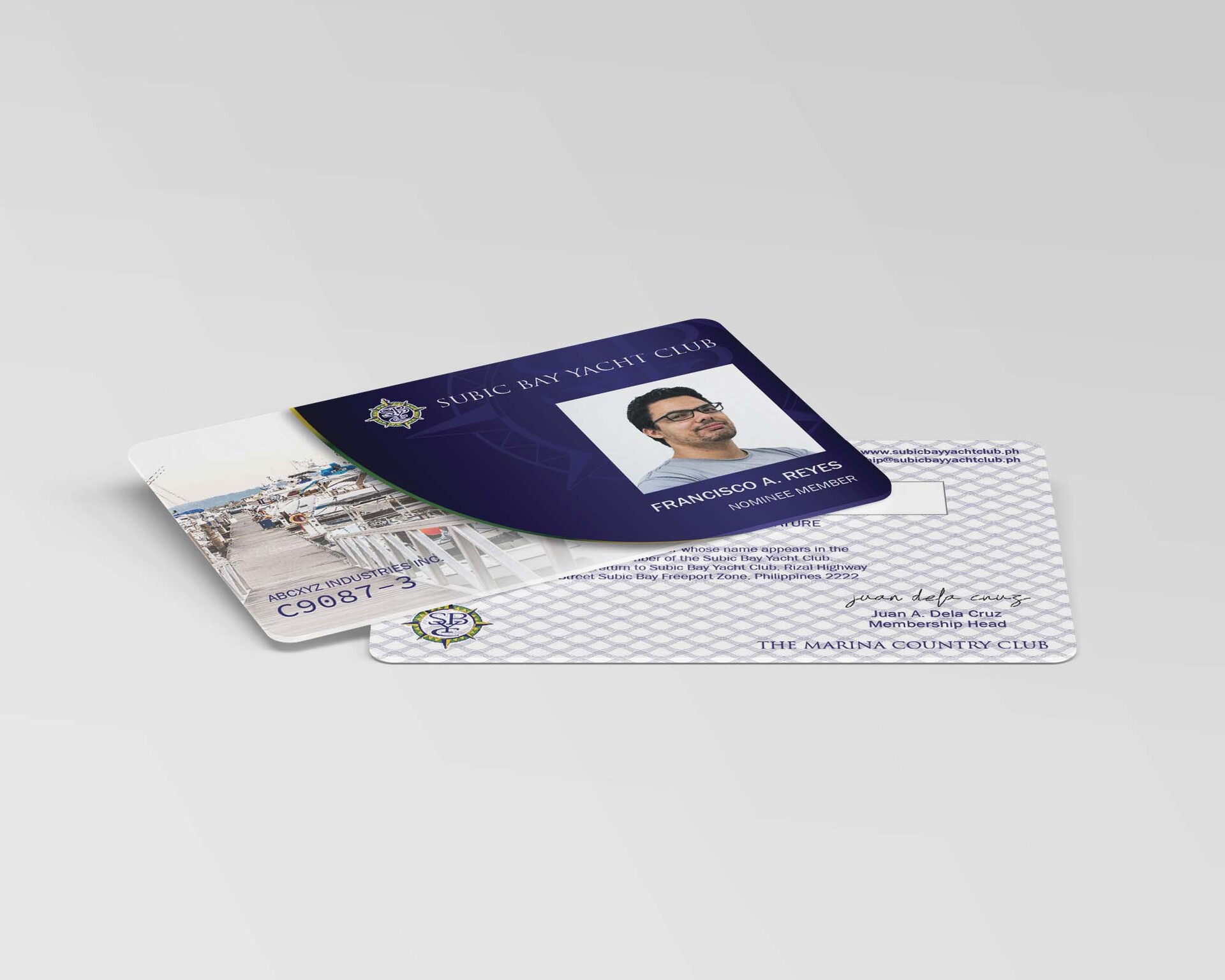The photograph features two identification cards set against a white background. The top card belongs to Francisco A. Reyes and identifies him as a nominee member of the Subic Bay Yacht Club. His portrait on the card shows a Hispanic male with dark hair, glasses, a slight beard, and wearing a blue shirt. The card includes an ID number in white text to the left, while the right side displays a photograph of yachts docked at a marina, indicative of the yacht club's location. The card also features a nautical logo.

The bottom card appears to be the reverse side of the same ID, with text stating "The Marina Country Club" and a symbol associated with the club. Below, it reads "Juan A. de la Cruz, Membership Head," in blue text, likely indicating the issuer or overseer of the memberships. The card likely includes an area designated for the member’s signature.